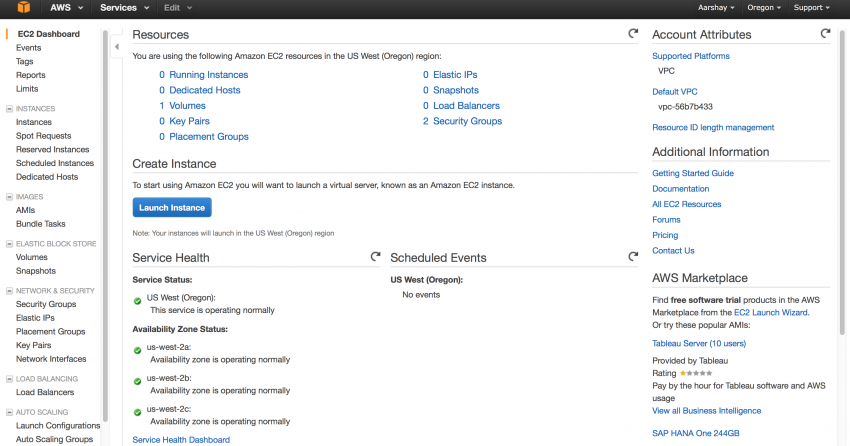This is a screenshot of an Amazon Web Services (AWS) management console window. At the top of the interface is a persistent black navigation bar, featuring the AWS logo prominently on the left. Adjacent to the logo, dropdown menus labeled "Services," "Edit," and other navigation options are available for quick access.

Directly below the navigation bar, the screen is divided into two primary sections. On the left, there is a vertical sidebar menu exhibiting various expandable options related to AWS services. 

In the main viewing pane on the right, the "Resources" section is currently active. The interface displays a message indicating that the user is utilizing Amazon EC2 resources specifically within the US West region. The text highlights that there are nine active resources, which are emphasized in blue to denote their current usage.

Additionally, there is a prominent, blue "Launch Instance" button within the "Create Instance" menu, allowing the user to quickly initiate a new EC2 instance. The layout and details provide a comprehensive overview of the AWS EC2 resources being used and offer accessible controls for managing instances.